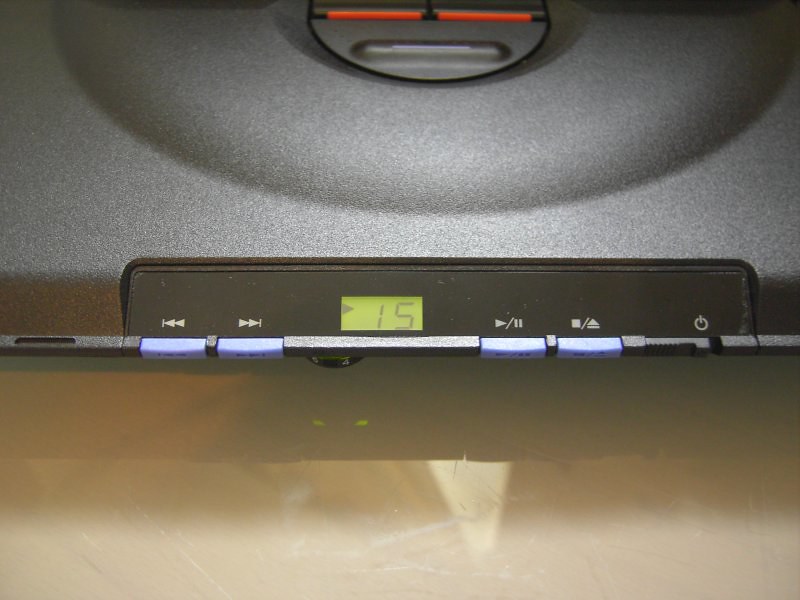This close-up photograph features the bottom half of a black and silver electronic device, identified as likely a CD player. Central to the image is a green, 90's era digital display showing the number "15", possibly indicating a track number. Surrounding the display are various buttons: blue fast forward, rewind, stop, and pause/play buttons are prominently visible. Additionally, there are an open/close button and a power button on the device. The design includes a rounded, plastic component, inferred to be the CD compartment. The device is partially reflected on the glass table it rests on, enhancing its sleek, modern aesthetics.